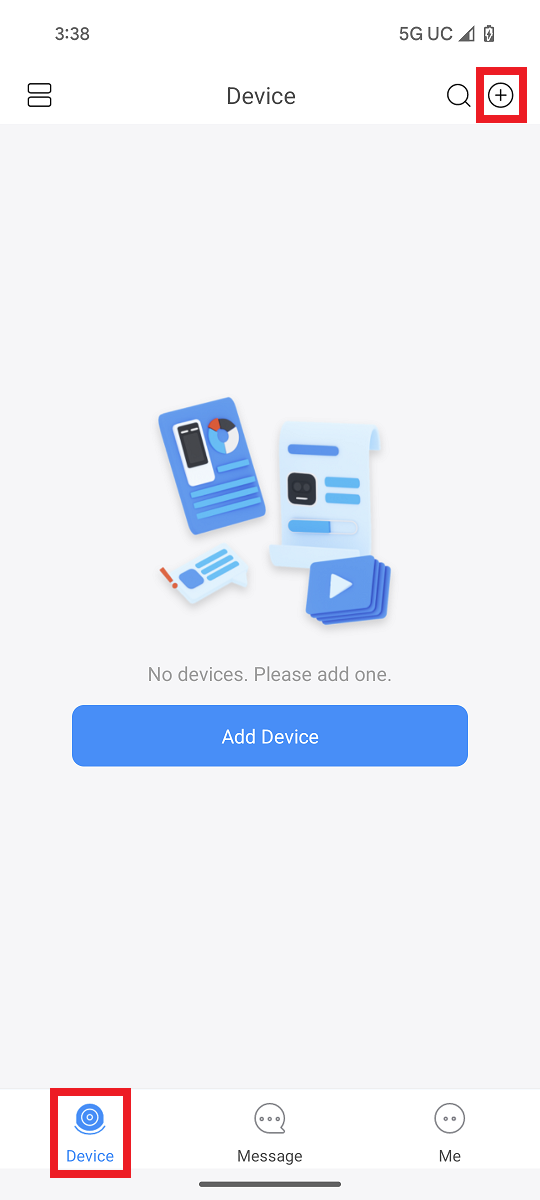The image displayed on a mobile device features a predominantly white top section, a light gray rectangle in the middle, and another white section at the bottom with a light gray band across the very bottom edge. 

At the top of the image, on the white background, the screen displays various elements: the number 3:38, icons for 5G UC signal, battery, and other status icons. Next to these, the word "Device" is visible, followed by a magnifying glass icon for search and a circular add icon. The add icon is prominently highlighted with a thick red square around it.

The central gray rectangle holds various blue, black, red, and white illustrations, predominately blue with minimal black and red accents. The illustrations depict a chat speech bubble, graphs, a smartphone, a scrolling document, and a play button. Text in this section reads "No devices. Please add one," indicative of no current devices being added to this interface. Below this message is a long, bright blue button with white text that says "Add Device."

At the bottom of the page, as it transitions back to white, there are three clickable options: "Device," "Message," and "Me." The "Device" option is currently selected, indicated by its blue coloration and a thick red square highlighting it.